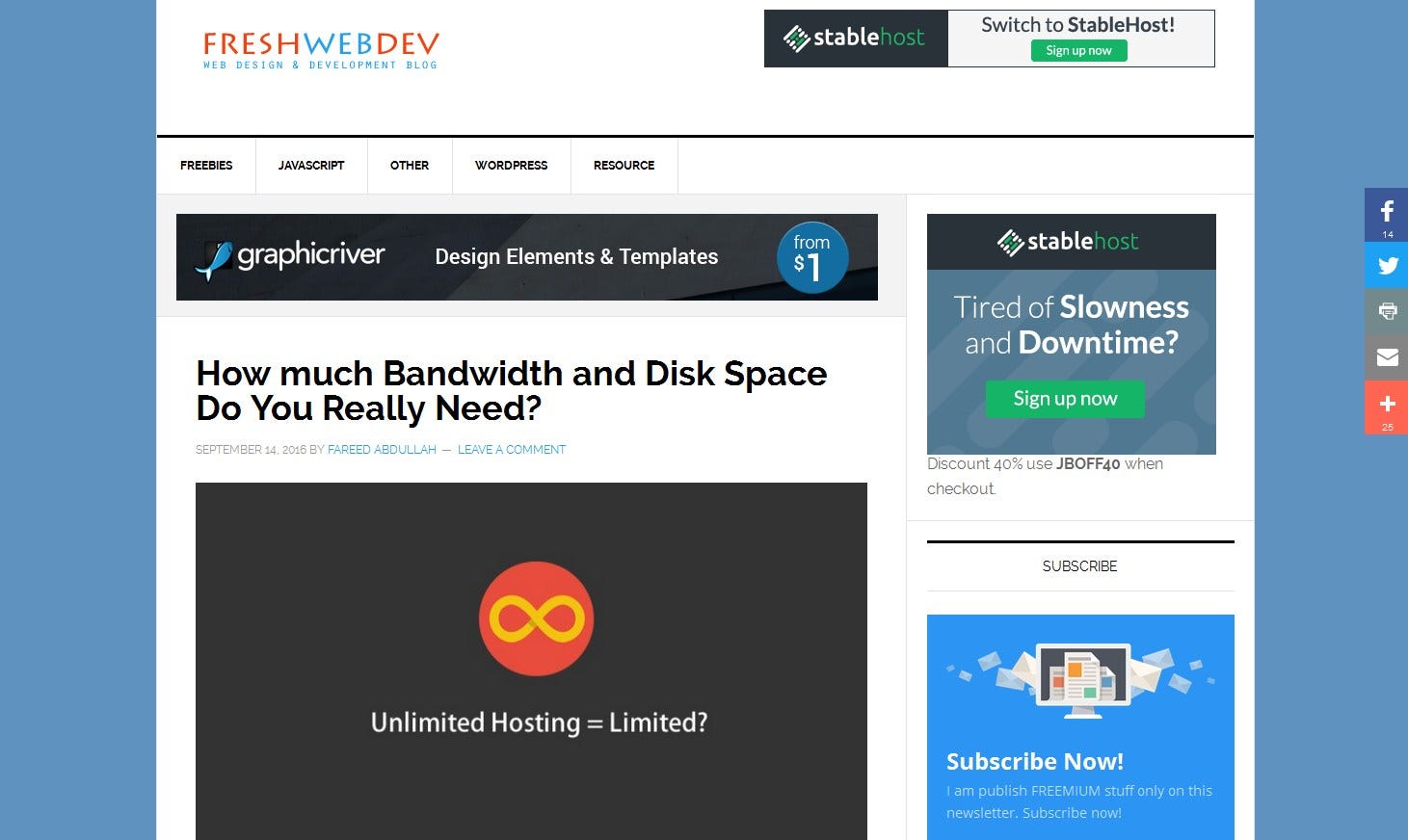This image is a screenshot of a web page featuring a header with a white background. In the upper left corner, the text "Fresh Web Dev" is prominently displayed; "Fresh" is in red font, "Web" is in blue, and "Dev" (spelled D-E-V) is also in red. Below this, the phrase "Web Design and Development" is written in blue font. Under the header, a line extends horizontally across the page, bordered by vertical blue blocks of color on either side, while the rest of the background remains white.

The navigational menu, written in black font, lists the categories: Freebies, JavaScript, Other, WordPress, and Resource. Below this, a black rectangle contains the text "GraphicRiver" (written as one word) in white, followed by "Design Elements and Templates." Adjacent to this text is a blue circle with the words "From $1" in white.

Further down, a headline against a white background reads: "How Much Bandwidth and Disk Space Do You Really Need?" Below this, a dark gray rectangle holds the text "Unlimited Hosting Equals Limited?" in white, with a question mark. Above this text, a red circle contains a yellow number 8.